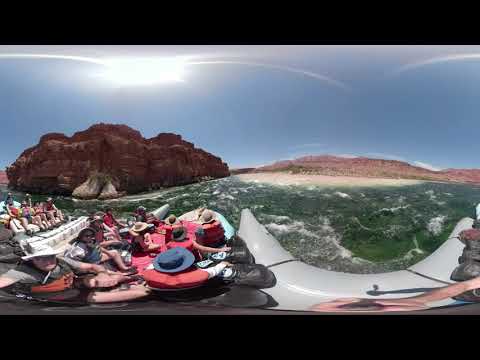This is a panoramic, 360-degree daylight image capturing a group of people navigating a vibrant green waterway, likely within a canyon setting, potentially the Colorado River. The image is presented with fisheye distortion, resulting in a slightly warped appearance, and is bounded by black bars at the top and bottom, suggesting it may be a still from a video. The scene is lively with numerous people onboard large gray rafts or pontoon boats, all adorned in red life vests and a variety of hats including white, blue, and brown, indicating a mixed group of men and women, potentially tourists.

The waterway beneath them is dynamic, frothing with waves and dotted with sea foam. Surrounding the water, to the right, stands a prominent reddish-brown rock outcropping, towering above a white sandy beach. On the left side of the image, more eroded and flattened rocky formations line the shore, adding to the rugged canyon landscape. The bright blue sky overhead is almost cloudless, accentuated by the large, intensely bright sun positioned in the upper left, appearing slightly stretched out due to the panoramic effect. This sunny day casts clear shadows of various items and emphasizes the hats and shorts worn by the adventurers, highlighting the vibrant outdoor scene.